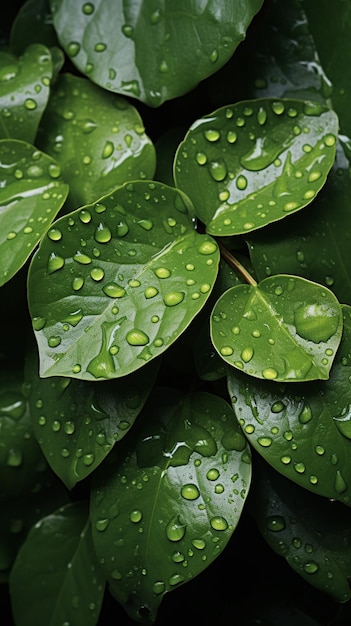This is a vibrant macro photograph capturing approximately fifteen bright green leaves with sharp tips, adorned with glistening water droplets. Against a stark black background, the image is twice as high as it is wide, offering a high-contrast view featuring shades of black, green, and white. The central leaves are well-lit, possibly by studio lighting, which adds a reflective shine and highlights the droplets, creating a shimmering effect. The edges of the image fade into darker, less distinct foliage, adding a sense of depth and artistic flair. This close-up shot, with some leaves curving upward and others downward, evokes a peaceful and dynamic atmosphere.